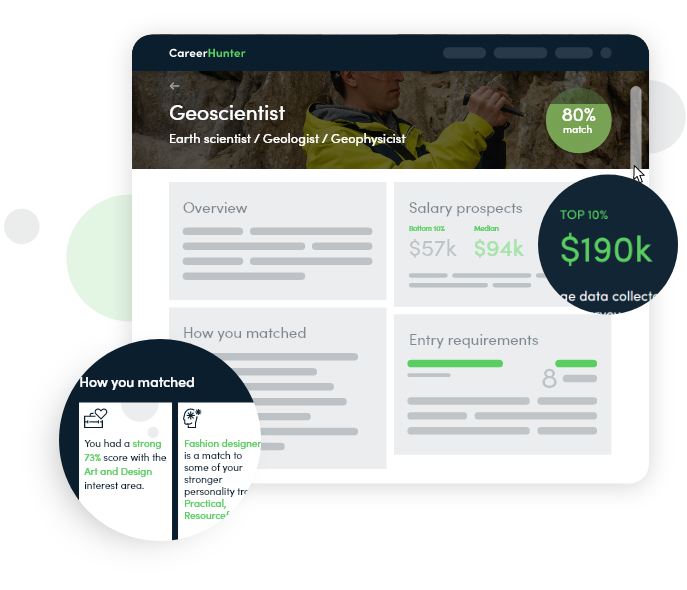The screen capture appears to be taken from a career advice website named "Career Hunter," as indicated by the black bar at the top with "Career Hunter" written in white and green text. Below this header, there are three gray boxes and a gray circle. 

The main section of the image features a photograph of a man wearing a yellow coat and safety goggles who is chiseling at a rock. Overlaying this image are white texts that read: "Geoscientist, Earth Scientist, Geologist, Geophysicist." To the left of this, there is a back arrow icon.

On the right-hand side, a green circle displays an "80% match" in white text. Below this, a white mouse cursor is pointing towards a black circle with green accents that reads "Top 10% 190k."

Further down, there are four vertically-aligned gray boxes labeled as follows:
1. "Overview"
2. "How You Matched"
3. "Salary Prospects" with a subtext listing the range as "57k to 94k" in green and gray.
4. "Entry Requirements"

To the right of these boxes, there are two additional informational sections:
1. A briefcase icon with a heart, indicating that you scored a strong 73% in the "Art and Design" interest area.
2. A person head icon with a star, suggesting that the role of "Fashion Designer" matches some of your stronger personality traits.

In the background, there are several gray and green circles, adding to the visual complexity of the interface. The layout and various elements suggest an interactive and personalized career exploration tool.